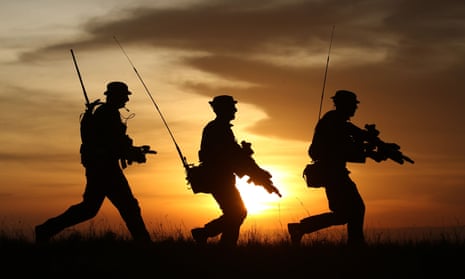The photograph is a full-color, rectangular image with its longest edges on the horizontal axis, capturing a dramatic sunset. The scene features three silhouetted men walking or jogging towards the right, all wearing caps that oddly resemble bowler hats. Each man is carrying a large gun and has a big pack on their back with tall antennas protruding from it, extending above their heads. The central figure appears slightly shorter compared to the other two, who are of equal height. All three have their left foot forward, with the first two men’s right legs in a similar position while the third man seems to be taking a larger stride. They're moving through a grassy field with vegetation reaching up to their shins, also silhouetted against the backdrop. The sky is moody with dark clouds and painted in shades of orange from the setting sun, casting an eerie, atmospheric light over the scene.